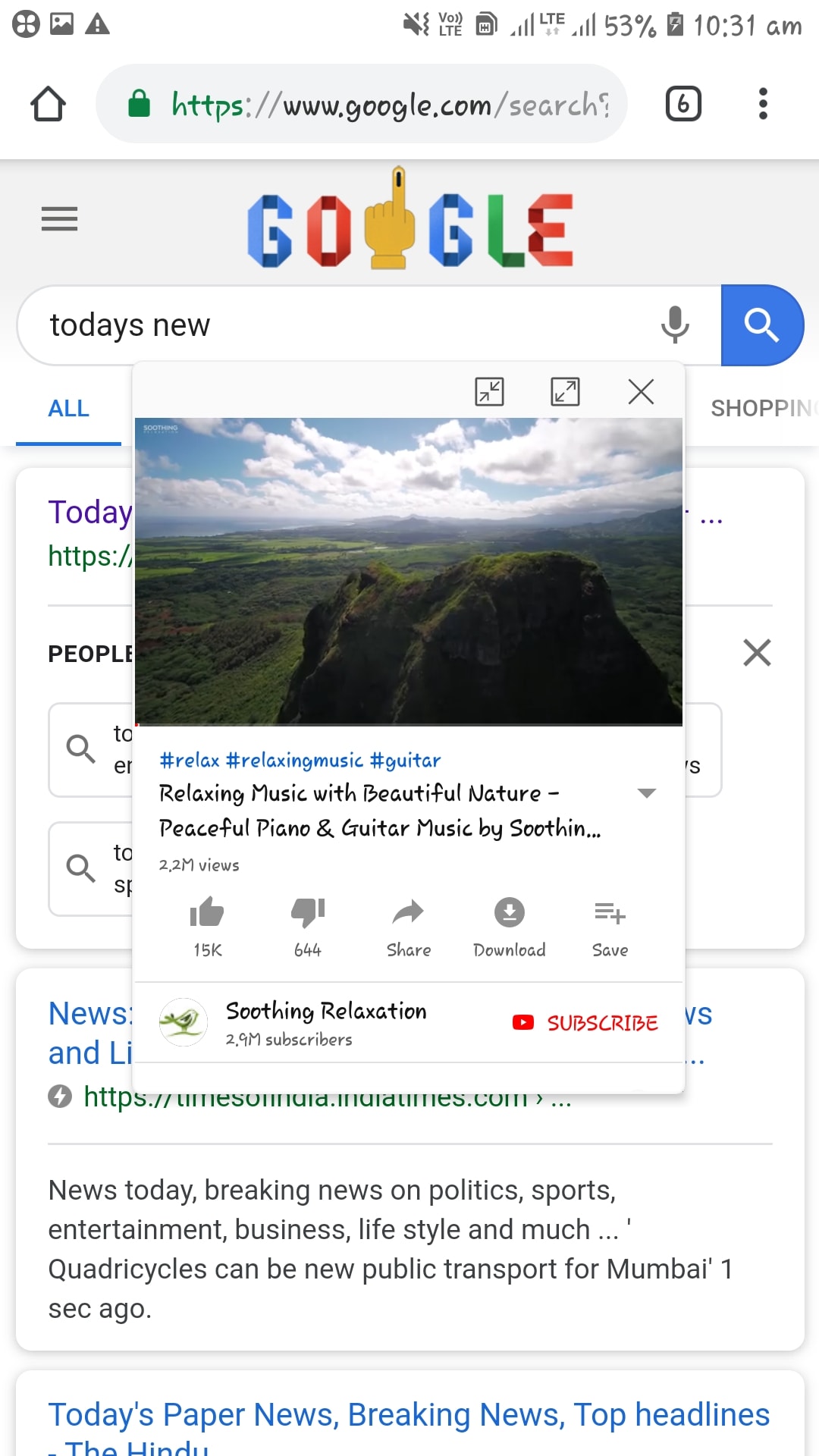This image is a detailed screenshot from a mobile phone, showcasing various interface elements and a Google search page. In the top left corner, the background is predominantly white, housing a circle logo with a white butterfly, a photo icon, and a triangle icon with a white exclamation point. Progressing to the right, the screen displays a muted speaker icon (indicated by a slash through it) followed by small gray text reading "VOD LTE". Next, an SD card icon and two mobile signal icons are visible. The battery percentage is noted as "53%" alongside a battery icon, with the time displayed as "10:31 AM."

Below this status bar, the main content of the screenshot is centered on an open Google search page. The URL bar clearly shows "https://www.google.com/" and indicates six other browsing tabs. Beneath the address bar, a darker gray rectangle features the colorful Google logo. Directly below this, a white search field prominently displays the text "Today's New" with a black microphone icon on the right and a blue half-oval housing a white magnifying glass icon on the far right of the search bar.

At the bottom of the image, there is a white square pop-up menu in the upper right corner that includes minimize, maximize, and close (X) icons. Within this pop-up, a photograph depicts a scenic mountaintop in a verdant area under a clear, blue sky.